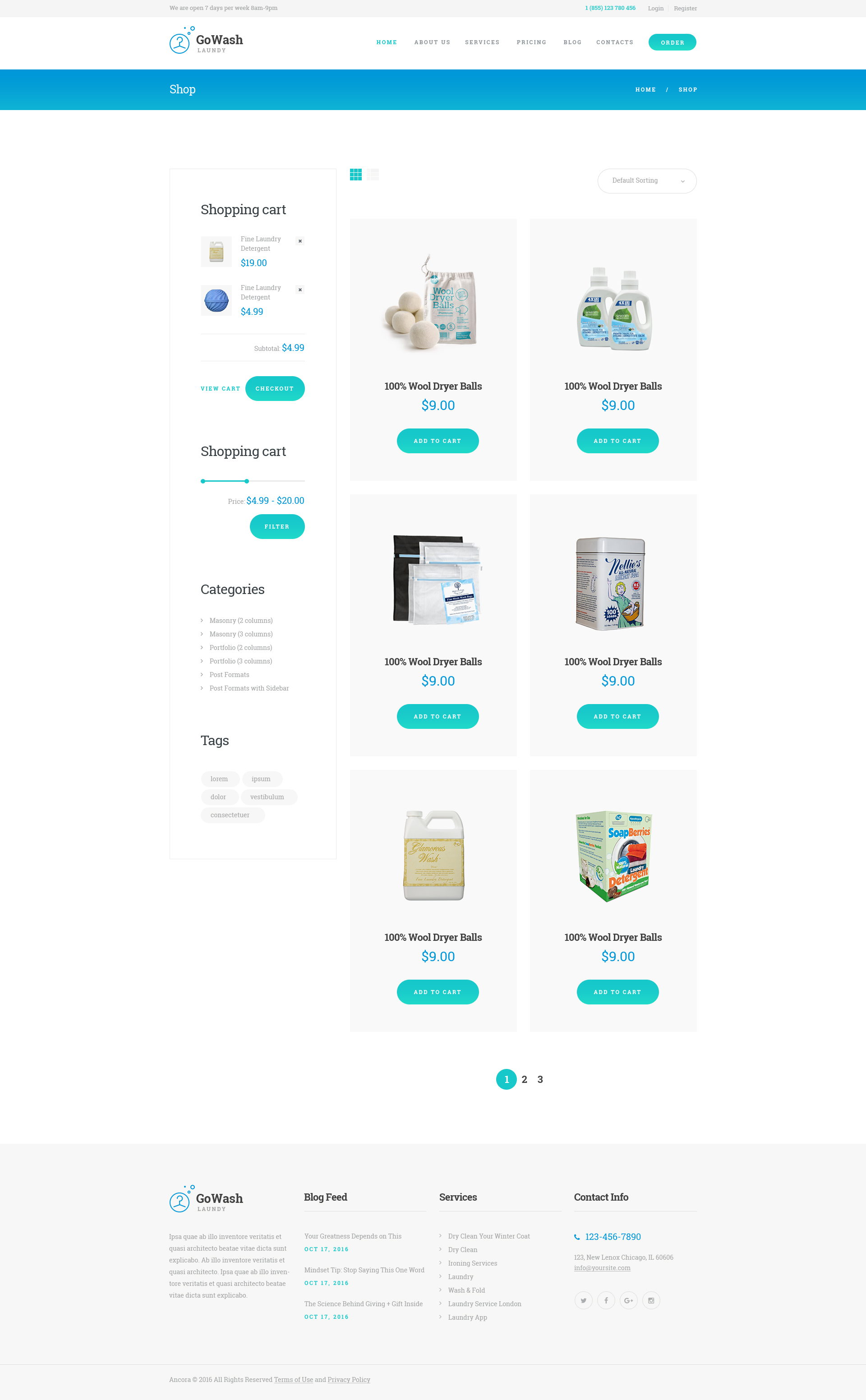The image is a low-quality screenshot of a webpage, making text largely unreadable. At the top, the background is white with an illegible menu and company name. The company name, rendered in black, seems to be a single word, accompanied by a logo that appears to be a blue circle, although the details are unclear.

Below the menu, there is a blue border in a shade close to turquoise, which is aesthetically pleasing. The rest of the page has a white background. This appears to be a retail site, as indicated by a sidebar on the left featuring shopping cart categories and tags, the only readable text on the page.

The main content area displays two rows of items, with four items in each row. In the upper right corner, there is an image that seems to depict two large containers of laundry detergent, possibly of the All brand. To the left of these containers, there are items that resemble garlic bulbs. In the lower-left corner, there is a large jug, which might also be a container of laundry detergent.